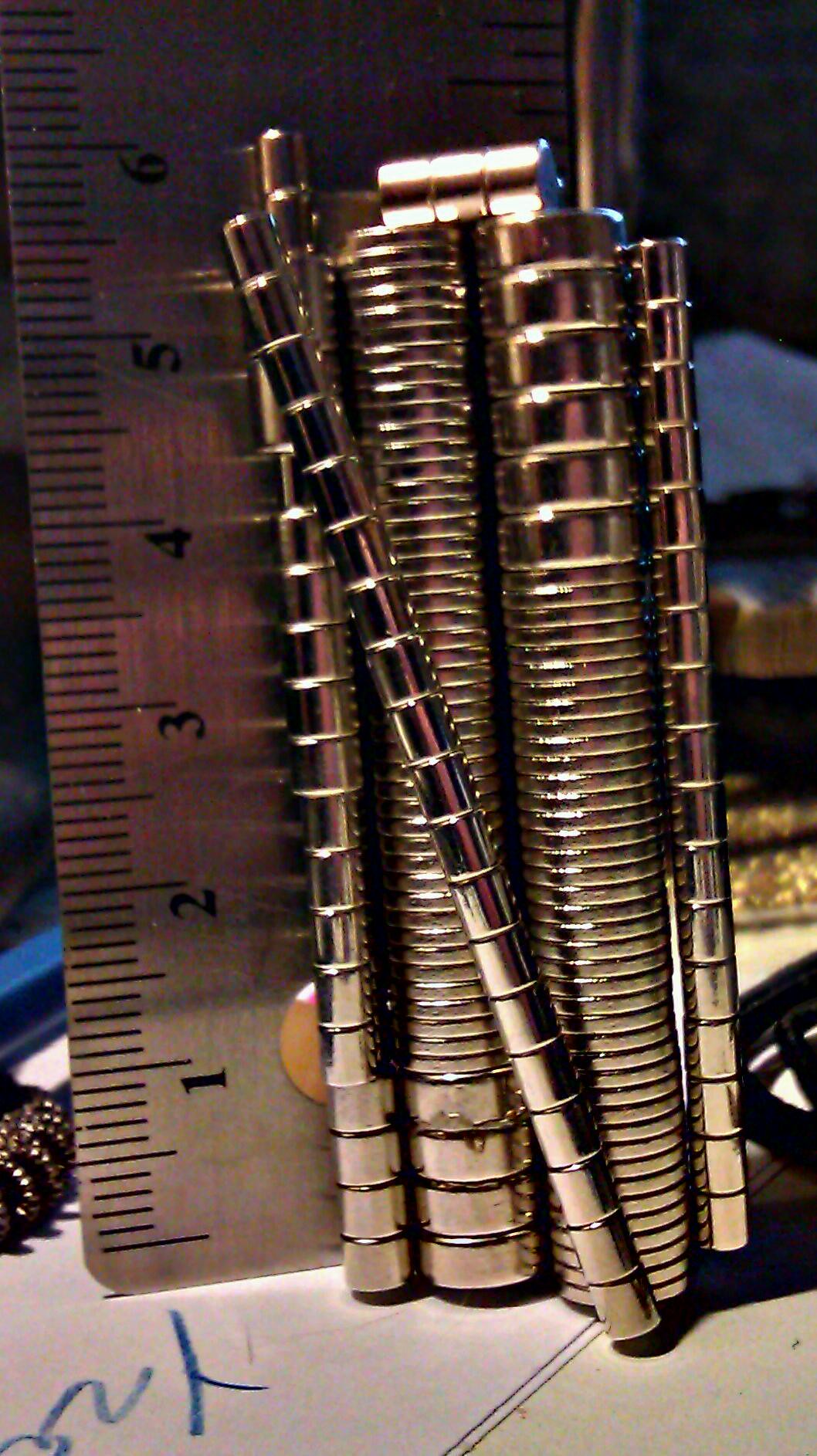This close-up image, likely taken on a desk or workbench, reveals a collection of precision tools. Dominating the frame is a wooden or brass metal ruler standing upright, displaying measurements up to around six inches. Adjacent to the ruler are several brass-colored, round threaded rods. These rods, resembling small magnets, are meticulously arranged, with variations in their ridges and grooves. Some have closely spaced grooves, while others have widely spaced ones, and they differ in diameter—some shorter and some larger, all generally between five to six inches in length. One of the rods appears to be leaning precariously, about to topple. The items are set against a white surface, which might be paper or a white board, featuring a blue pen marking that appears to read "Y2." In the background, a scattered assortment of hand tools and additional papers suggests a workshop setting utilized for intricate repairs.